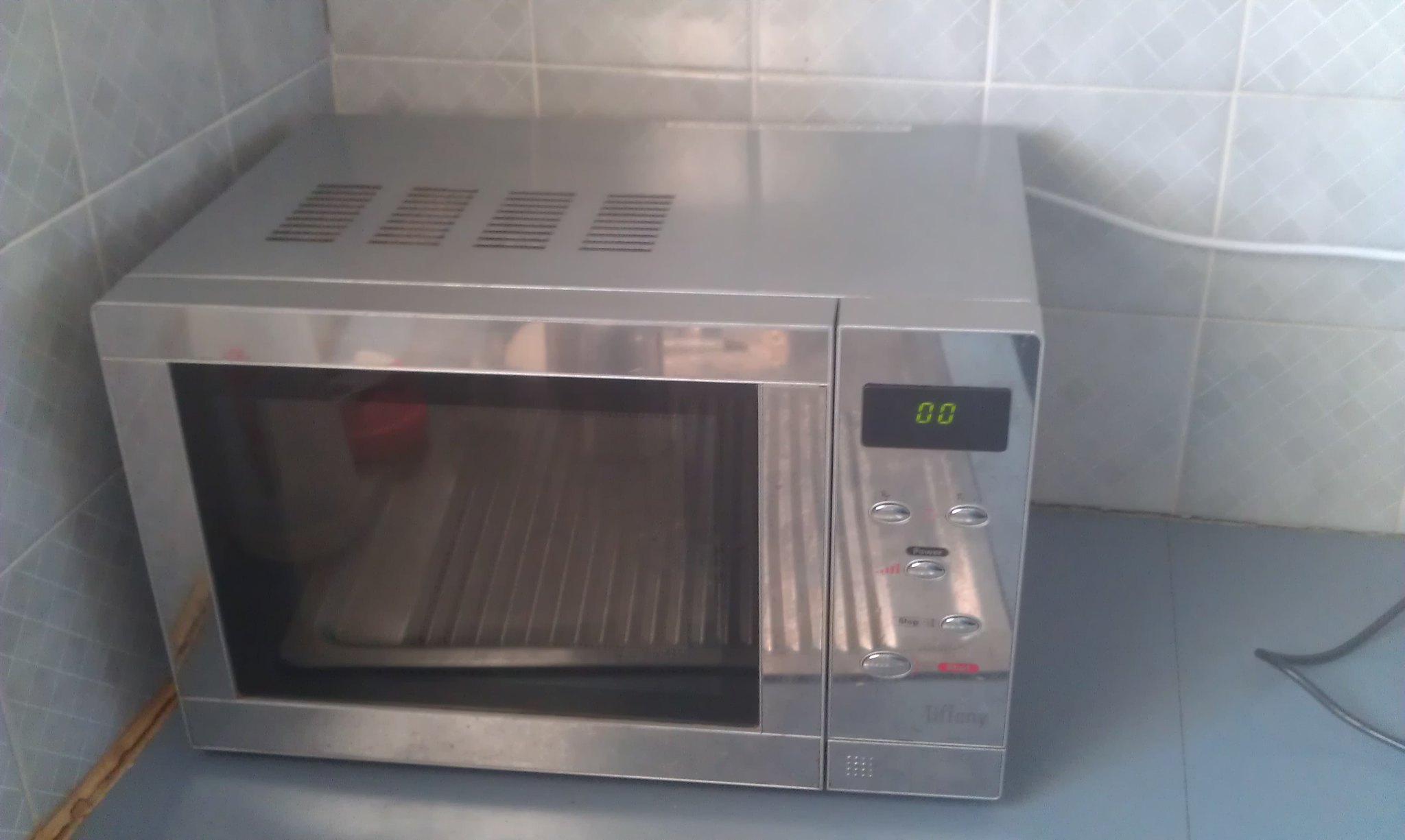The image features a close-up shot of a simple, metallic silver microwave oven situated in a left-hand corner. The front of the microwave includes a black window and a digital display panel on the upper right, which shows "00" in lighter green numbers. The panel is surrounded by five buttons, though only the "power" button in the middle is legible. Beneath these buttons is the brand name "Tiffany" in very light text. The microwave's black plug extends to the right side. It rests on a light blue countertop made of tile, contrasting with the gray tiled walls that feature a white checkered grout pattern. Additionally, there is a white cable to the right of the microwave, likely for power, and a gray cable in the bottom right corner of the image. The metallic surface of the microwave reflects an unidentified metallic object in front of it. The top of the appliance includes ventilation grates for air circulation.